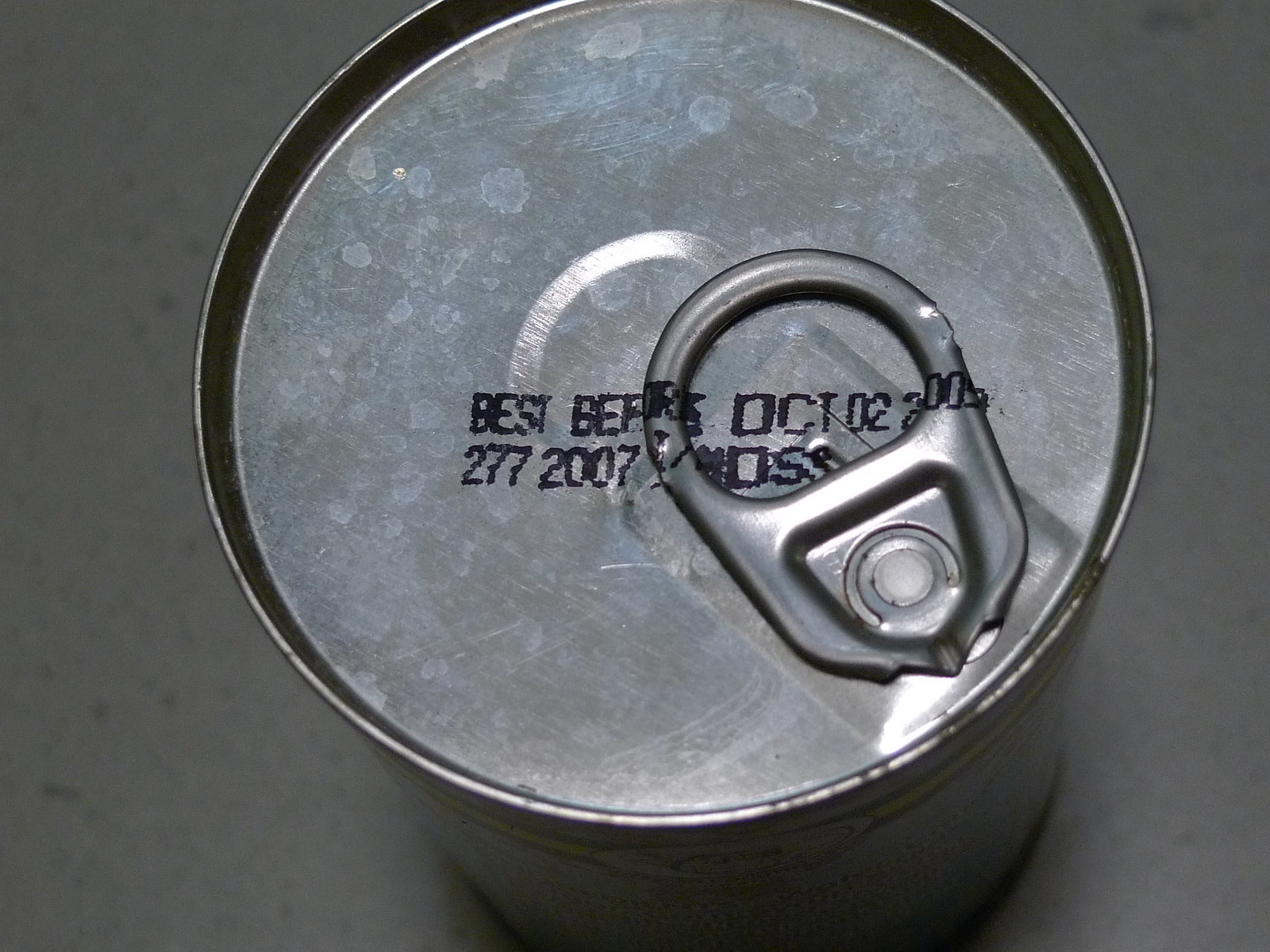This image captures a slightly aged tin can viewed from the top down, placed on an off-white, lightly speckled, marbled countertop. The can is primarily composed of steel or aluminum and features a pull-tab lid, which is slightly twisted to the right rather than sitting flush as intended. The label of the can, mostly out of view due to the angle, has a visible yellow border and possibly a company symbol. The top of the can is marked with a "best before" date stamp, reading "October 02, 2005," though part of the date is slightly cut off, showing only "200." Underneath the date, the identification number "277-2007 MOSS" is printed in black. The metallic surface exhibits a patina with fingerprints and light scratches, indicating some wear and age. The lighting suggests the photo was taken in dim conditions, possibly in the afternoon, with the flash providing the primary illumination.